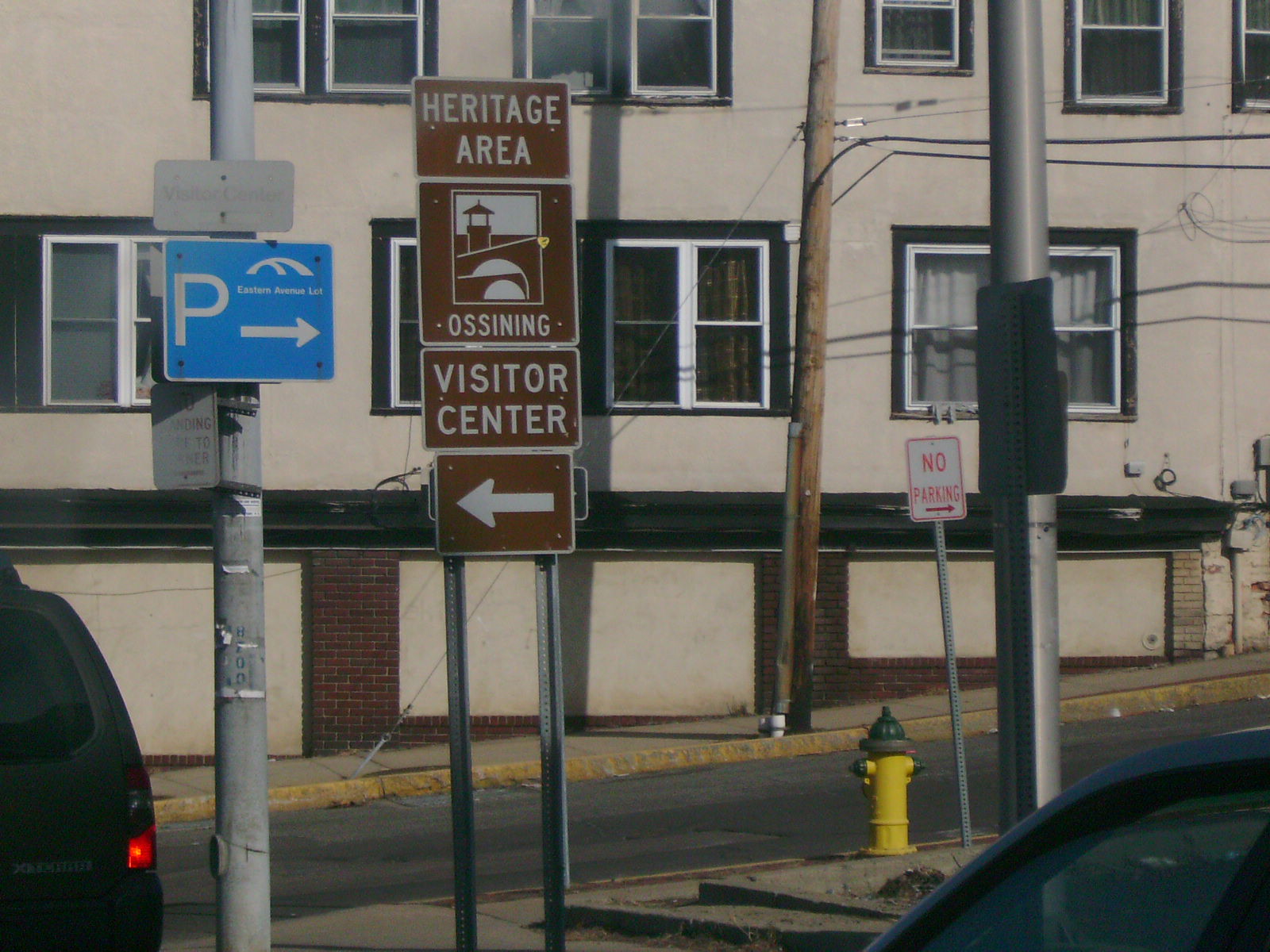This image, captured from the window of a moving car, showcases an urban scene, potentially in a city or town center. The focal point is the array of tall, tan-colored buildings adorned with brick facades at their base and numerous windows on the upper floors. In the foreground, the bottom left corner depicts the edge of a parked car, while the bottom right corner features the window of another vehicle, suggestively parked. Dominating the middle of the frame is a sign mounted on a brown post, indicating the direction to the Heritage Area and Ossining Visitor Center, with an arrow pointing left.